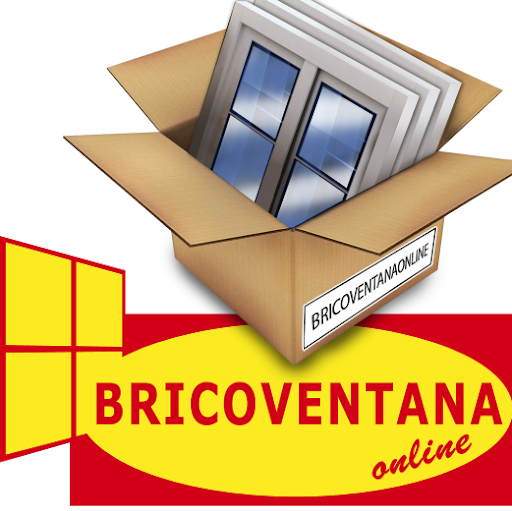The image is a highly detailed, cartoon-like or computer-generated depiction of an open cardboard box. The box, positioned prominently in the center of the upper half of the image, contains three slightly slanted window panes stacked inside. These windows have sleek, gray metal frames dividing each into four blue-tinted glass panels with a horizontal bar splitting each panel into two sections. The cardboard box is light brown and features a white label on its side with the text "BRICOVENTANAONLINE" in black letters and a black border.

Below the box, occupying the lower section of the image, is a vibrant logo. This logo consists of a red rectangle housing a yellow oval. Inside the oval, the word "BRICOVENTANA" is displayed in bold red capital letters, with "ONLINE" written in red script slightly offset to the right below it. To the left of this text is a graphic resembling a four-paned window, with yellow sections bordered by a red frame.